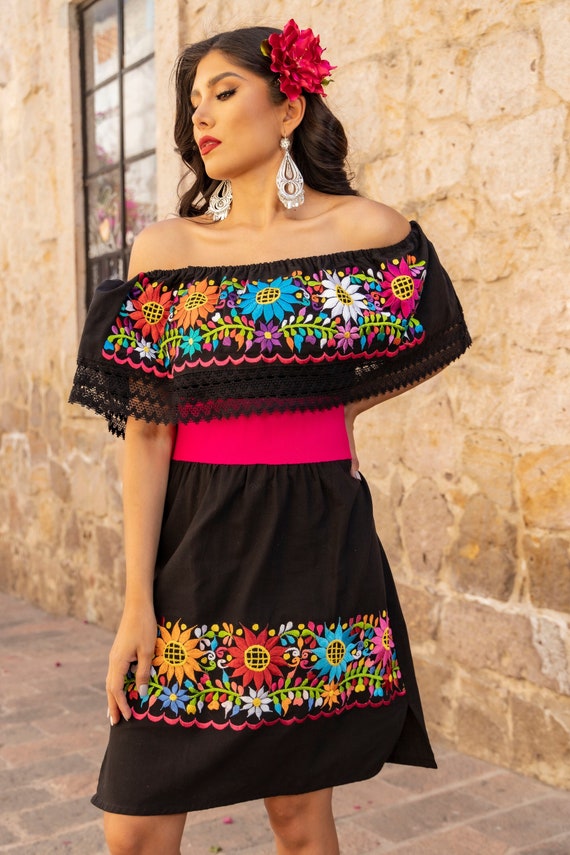The photograph captures a young Latina woman of likely Mexican heritage, standing gracefully in front of a beige stone building with a window that features a dark brown frame and multiple panes. She is adorned in a black off-the-shoulder dress, highlighted by vibrant, multicolored flowers—red, orange, blue, white, and pink—arranged across the bodice and again at thigh level on the skirt. The dress also features decorative pink stitching and lacy frills underneath. A wide red belt cinches her waist, complementing the large red flower nestled in her dark brown hair. She accessorizes with strikingly large silver earrings. In the photograph, she stands on a beige stone walkway, with her right arm resting along her side and her left arm bent at the hip, emanating a poised and elegant demeanor.